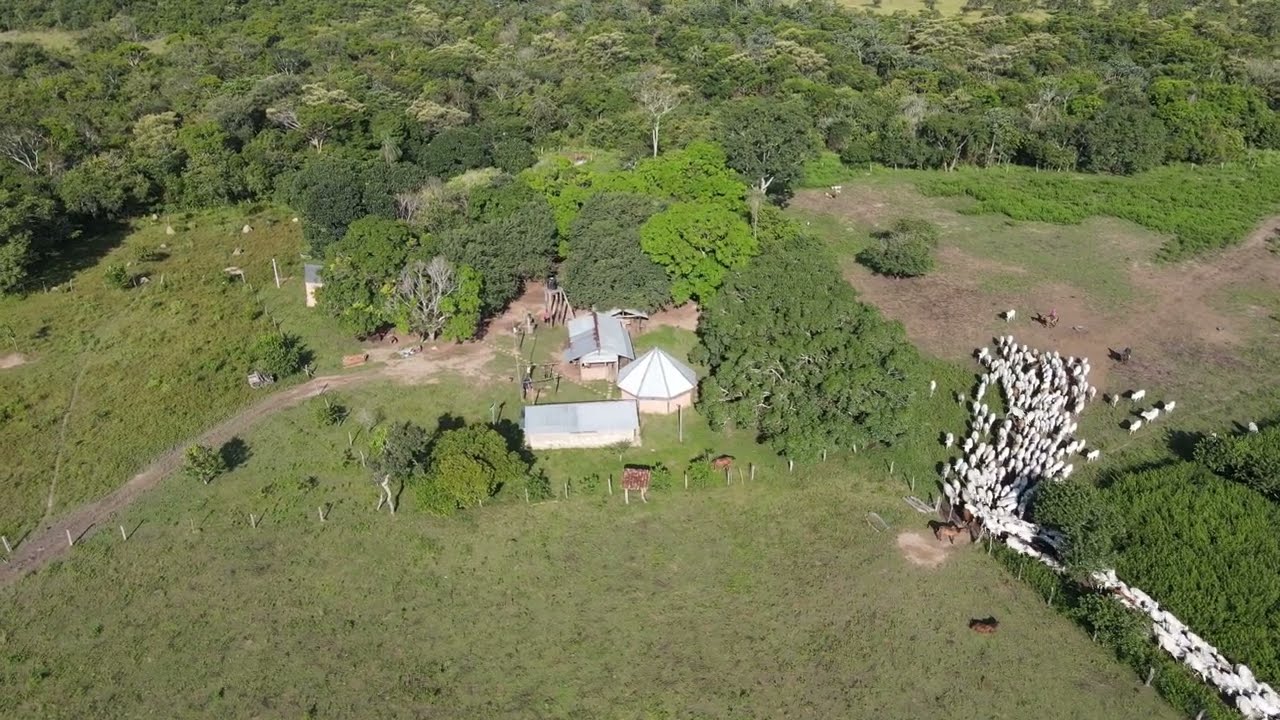This color, landscape-oriented photograph taken from a drone captures an aerial view of a countryside farm in the early evening. Central to the image are three main buildings, each with gray or silver metal roofs. The rightmost building is round with a segmented roof, resembling a grain bin, while two rectangular buildings are also visible, one of which appears to be a house. Surrounding these structures is flat land, sectioned by fencing and intersected by a dirt path on the left side of the image. To the right, a pasture hosts a mix of white sheep, some brown ones, and possibly a dark-colored dog, all moving towards a narrow pathway adjacent to a gate or fence. Shadows cast by the fence posts and animals confirm the early evening setting. The background features a dense forest, enhancing the overall picturesque and realistic representation of this tranquil farm scene.